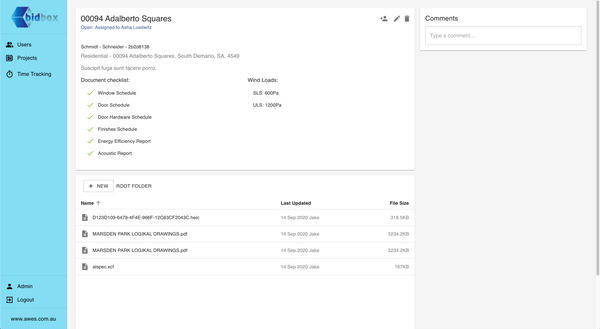The screenshot displays a section of a website featuring a prominent light blue-green colored rectangle titled "Bid Box" along the left-hand side. Under the "Bid Box" heading, there are several subsections listed in order: "Users," "Projects," and "Time Tracking." Below these options, clickable buttons labeled "Admin" and "Log Out" are clearly visible.

In the central part of the screen, a segment named "Open Assignments to Asha Schmidt" is highlighted. Further down in this area, a "Document Checklist" section is meticulously detailed, listing several categories, including "Window Schedule," "Door Schedule," "Door Hardware Schedule," "Finishes Schedule," "Energy Efficiency Report," "Acoustic Report," and "Wind Loads." Each category in the checklist from "Window Schedule" to "Acoustic Report" is marked with a single green checkmark, indicating completed or verified status.